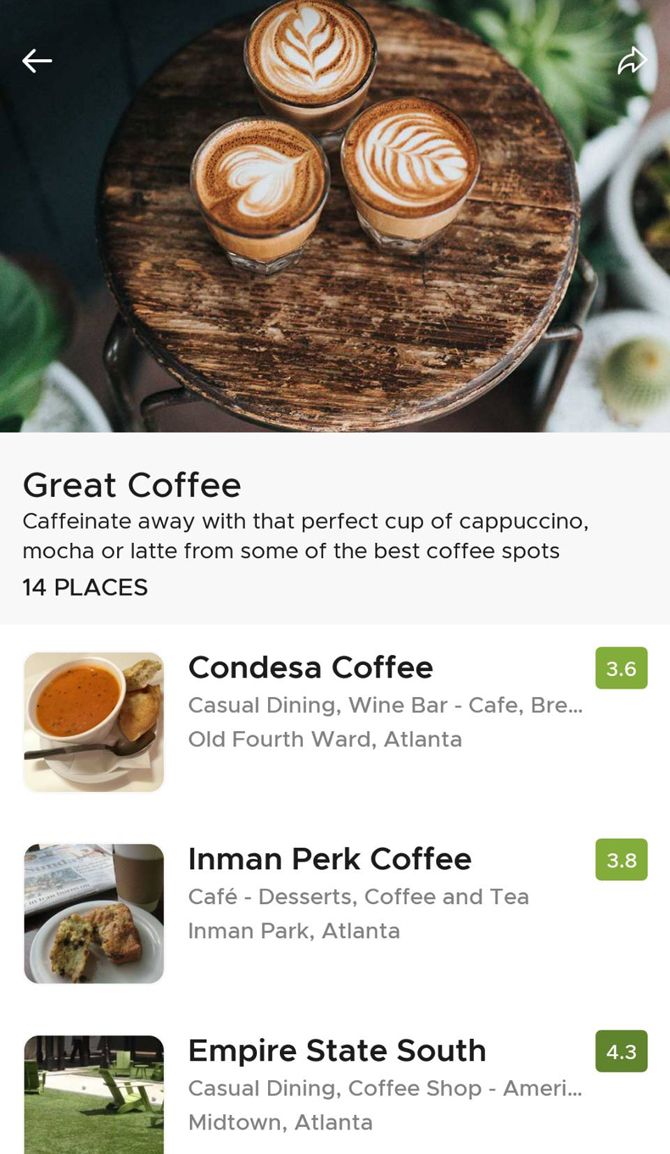The image features a pristine white background with a stylish wooden table supported by metal legs. On the table are three artfully crafted cups of coffee, each showcasing intricate latte art. The first cup displays a delicate leaf design, the second features dual leaf patterns, and the third shows a charming heart shape. These cups represent the diverse coffee offerings available, perfect for any coffee enthusiast looking to caffeinate with high-quality cappuccinos, mochas, or lattes. 

Additionally, several coffee spots are highlighted:
1. Inman Perk Coffee Cafe in Inman Park, known for its delightful desserts, coffee, and tea, boasting a 3.6 rating (indicated in a green rectangle).
2. Inman Park, Atlanta, with a 3.8 rating.
3. Empire State South, a casual American dining coffee shop located in Midtown Atlanta, with an impressive 4.3 rating. 

These establishments promise a great coffee experience in Atlanta.